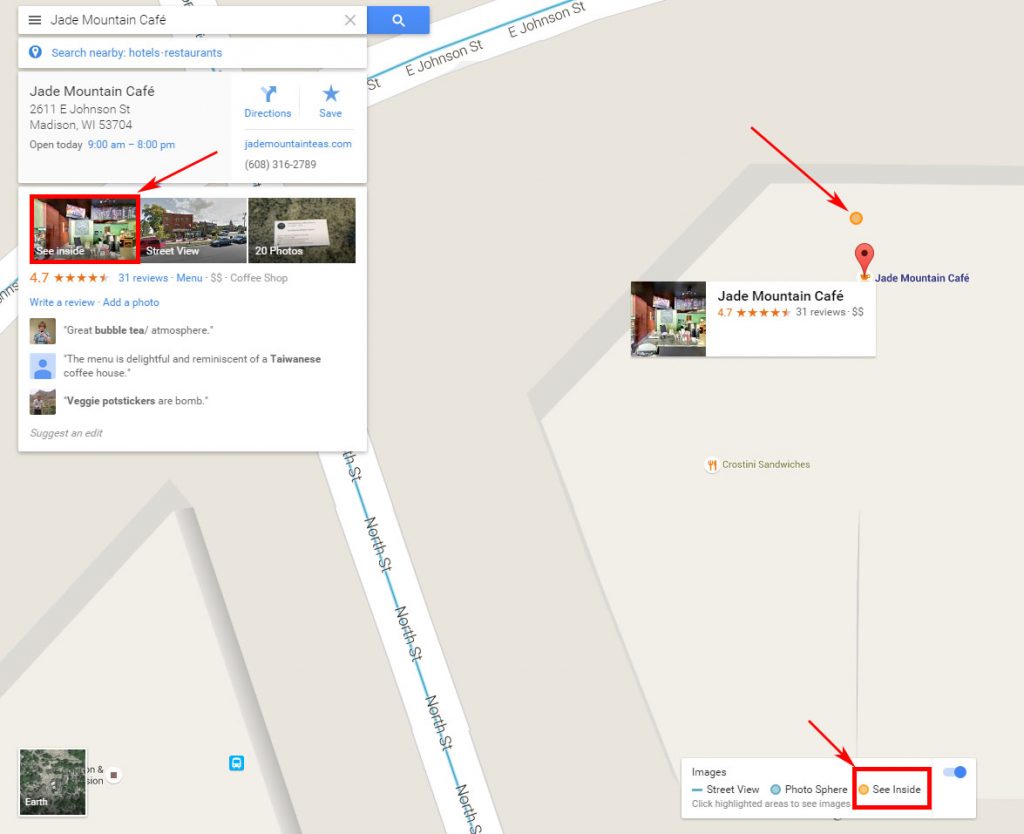The image features a detailed map highlighting the location of Jade Mountain Cafe, situated at 2611 E. Johnson Street, Madison, WI 53704. The map pin distinctly marks the cafe's position. Accompanying the map is information about the cafe's operating hours, which are from 9 AM to 8 PM. Additionally, the image includes options to view the interior, explore the street view, and browse through 20 photos of the establishment.

User-generated reviews are also visible, praising various aspects of the cafe. Highlights include commendations for the bubble tea, the inviting atmosphere, and a menu that evokes the charm of a Taiwanese coffeehouse. Specific menu items like the veggie pot stickers receive high praise, with one review describing them as "bomb."

The cafe boasts a high rating of 4.7 stars based on 31 reviews. Alongside this, there are suggestions for editing the listing, as well as prompts for users to write their own reviews or add photos. On the right side of the image, the street and nearby areas are depicted, with a note indicating the presence of crostini sandwiches in the vicinity.